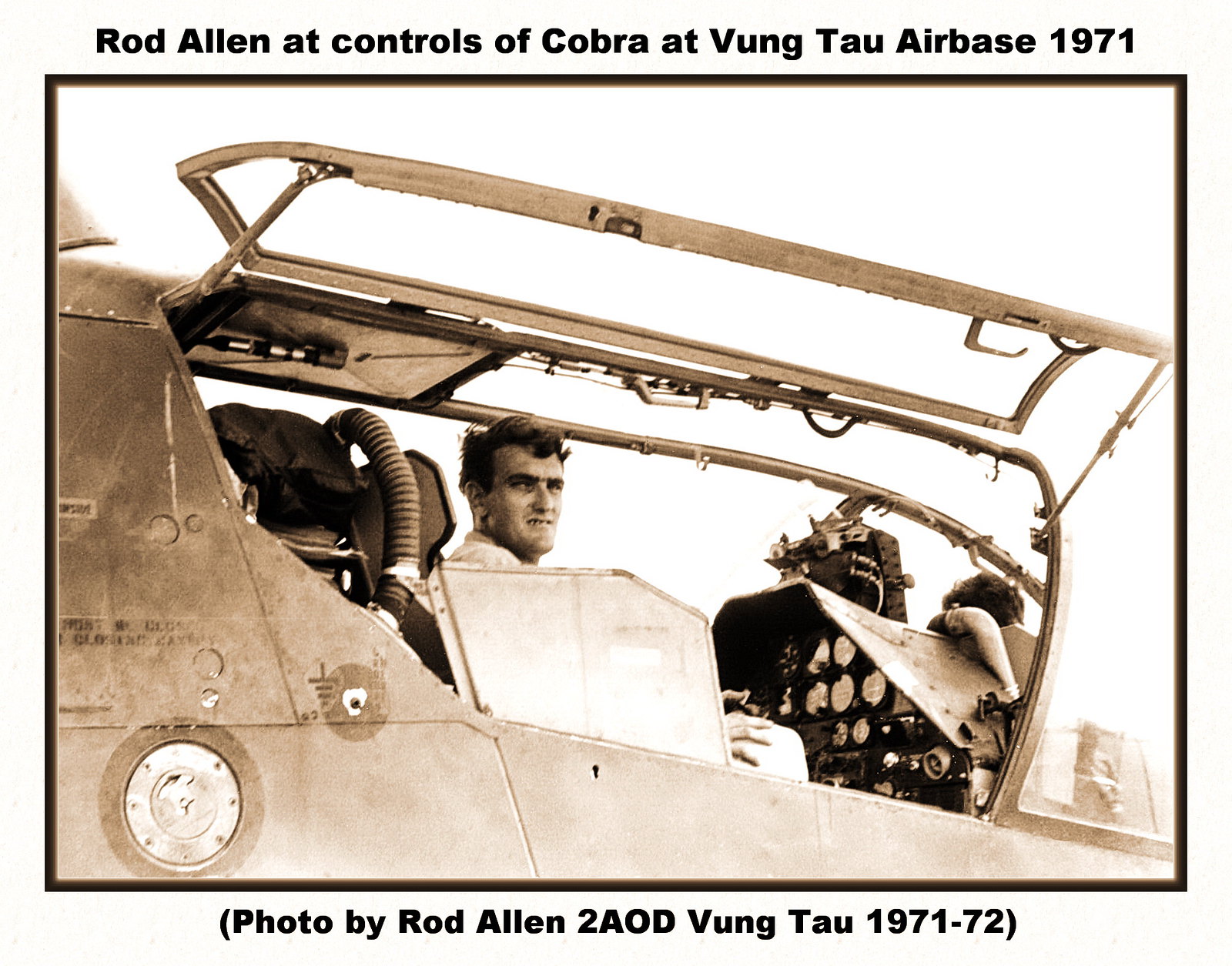This aged, sepia-toned photograph captures the image of a man, presumably Rod Allen, seated at the controls inside the cockpit of a Cobra attack helicopter at Vung Tau Air Base in 1971. The man, who appears to be a white male with dark, messy hair, is deeply focused with a stern expression, his demeanor suggesting the weariness of war. One hand rests on his knee while the other is near the controls. The helicopter's side window is open, revealing a glimpse of the aircraft's interior, including dials, gauges, and indistinct machinery extending behind him. The photograph, taken from the tarmac, includes a white border with bold black text across the top and bottom that reads: "Rod Allen at Controls of Cobra at Vung Tau Air Base, 1971" and "Photo by Rod Allen, 22nd AOD, Vung Tau, 1971-1972," indicating it is likely part of a personal collection from the Vietnam War era.